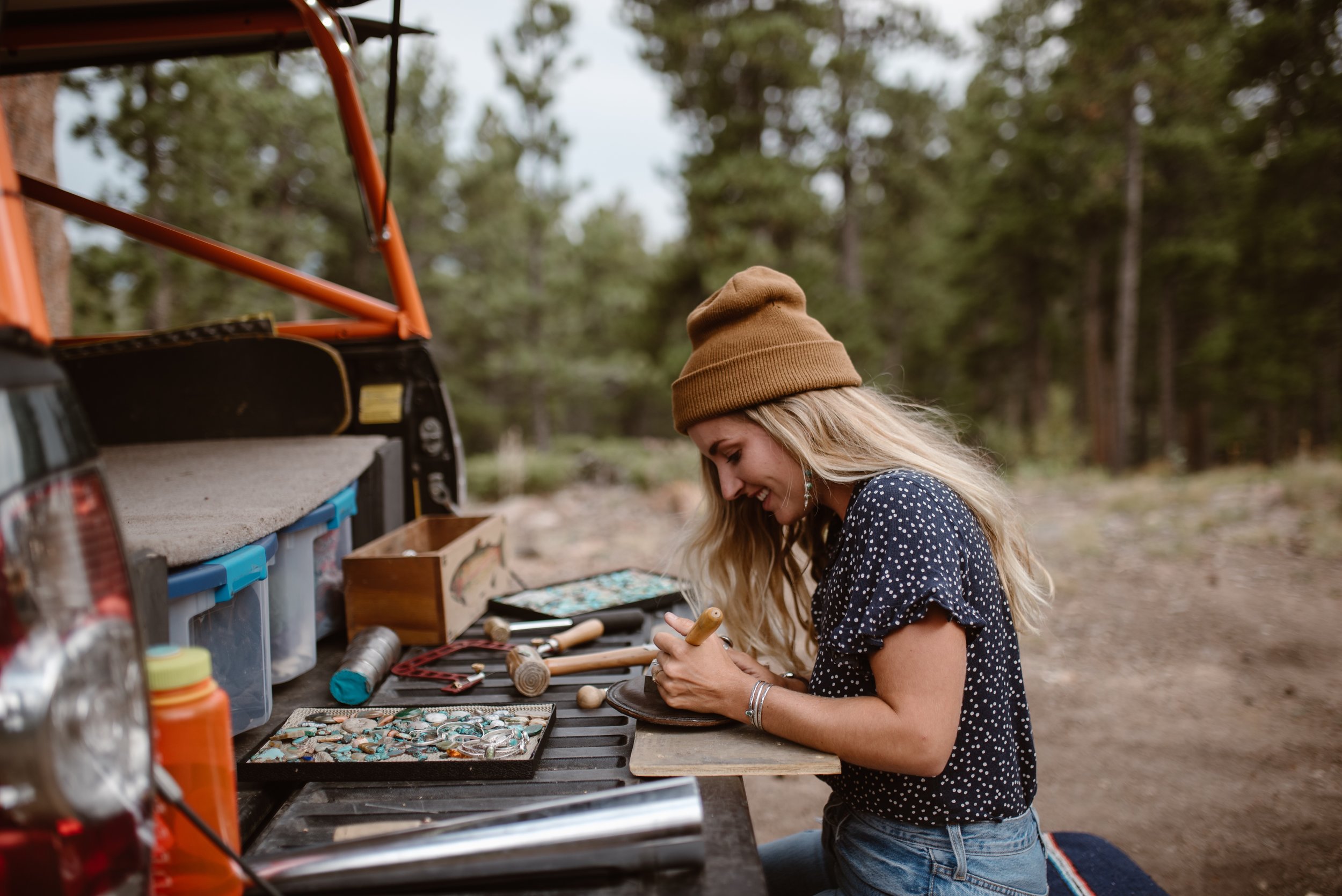A horizontal photograph captures a serene outdoor morning scene featuring a young Caucasian woman with long blonde hair working out of the back of a black pickup truck, which has its tailgate folded down. She's wearing a brown beanie, long silvery dangly earrings, and a short-sleeve black ruffled shirt with white polka dots, along with blue jeans. A silver bracelet adorns her wrist. The woman, who has a cheerful expression, is holding a tool in her left hand, suggesting she is engaged in some form of crafting or jewelry-making. The tailgate is scattered with various tools and bins, and there's an orange roll cage visible on the back of the truck. The background is slightly out of focus, featuring a worn-out field with some dirt and numerous evergreen trees under a pale blue morning sky.